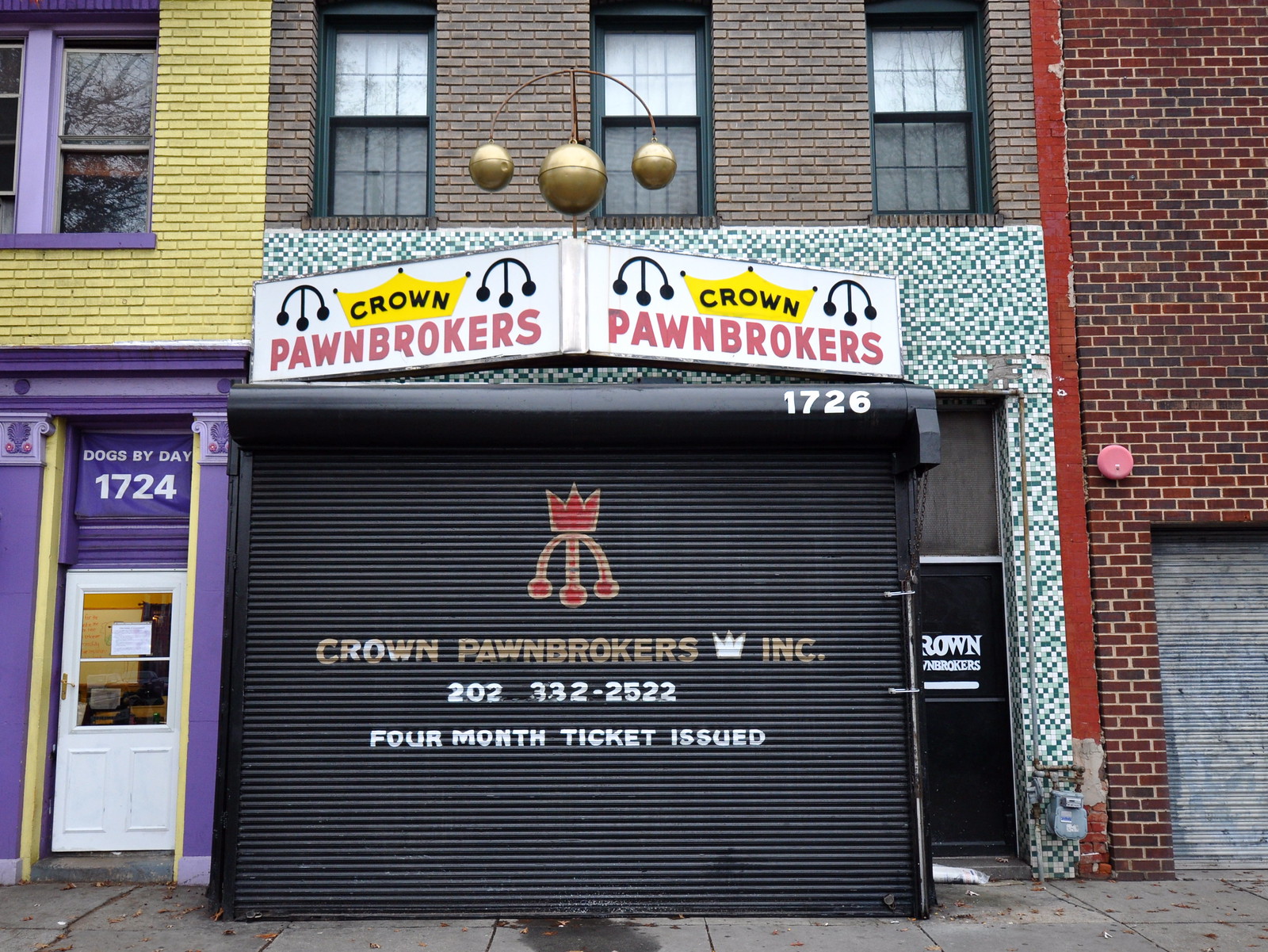The image showcases the front of a multi-story building with distinct sections made of different colored bricks: yellow with purple accents on the left side, muted brown in the center, and red on the right side. The central part of the building prominently features the storefront of "Crown Pawn Brokers." Above the storefront is a large sign with the business name and logo—depicting a crown—visible from both sides. The sign background includes green and white small checkered tiles. Below the sign, there is a metal garage-like door painted black with "1726" in white above it. The door also displays the text "Crown Pawn Brokers Inc.," the phone number 202-332-2522, and a note about issuing a four-month ticket. The left side of the building houses another store, indicated by a sign in purple and the words "dogs by day" with the address 1724, a white door with glass windows beneath it. The upper part of the central building has three windows with closed white curtains. The entire facade is unified by its brick construction, yet each section distinctly stands out due to the variance in brick color and design elements.